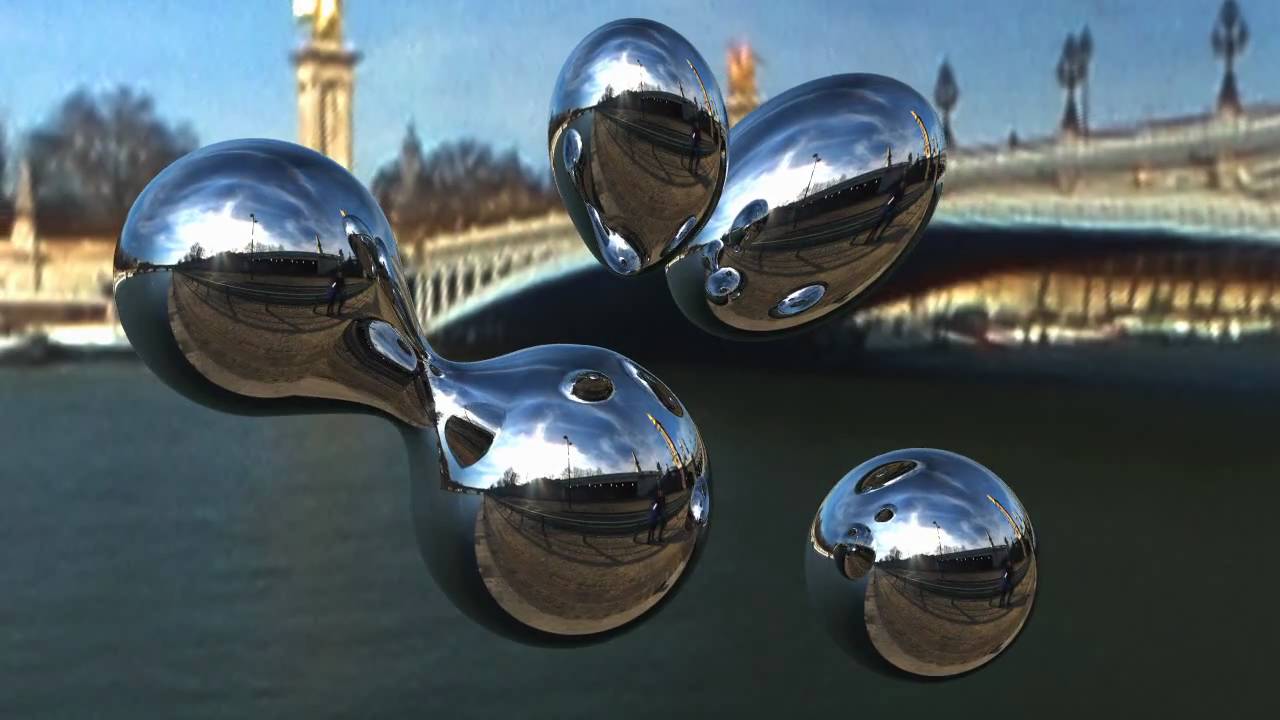This image captures an array of metallic, highly reflective ornaments that hang suspended in the air. Prominently featured on the left is a piece shaped like a tilted bowling pin or curved hourglass, angled around 45 degrees to the left. Centrally, two cylindrical ornaments and another rounded object sit adjacent to each other, reflecting their surroundings. Down at the bottom left corner lies a circular item. All of these pieces have a smooth, chrome-like finish that mirrors the background vividly.

In the backdrop, a dark blue body of water is visible, over which spans a white bridge accompanied by tall, white statues and columns. The sky overhead is a serene blue, giving a contrasting backdrop to the grayish-blue water beneath. A white building perches in the left corner, and distant trees as well as the suggestion of roads and streets add further context to the scene. The entire composition offers a blend of natural and man-made beauty against the striking metallic forms.